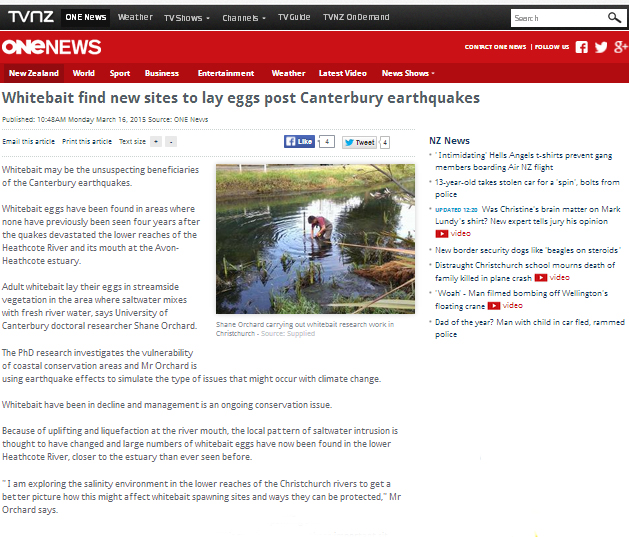The news webpage features a prominent black header with a dark gray left side and bold white text reading "TVNZ". Adjacent to the logo are several tabs, with the "One News" tab highlighted in black, contrasting the gray status of the others. The tabs include options for "Weather," "TV Shows," "Channels," "TV Guide," and "TVNZ On Demand." Below the header, a white bezel transitions into a red banner displaying "One News" in white text, marking the website title.

On the top right, clickable areas are available for contacting "One News" and following on social media platforms like Facebook, Twitter, and Google Plus. Beneath this, a news section is presented, with "New Zealand" selected and highlighted in dark red with white text. Other sections listed include "World," "Sport," "Business," "Entertainment," "Weather," "Latest Video," and "More Shows," the last accompanied by a downward arrow for more options.

Further down, an article headline in blue text reads: "Whitebait find new sites to lay eggs post Canterbury earthquakes." The accompanying image shows an individual wading in water, clad in gray waders and a pink short-sleeve shirt. The setting is a pond surrounded by green plants, some tinged brown. In the background, mixed patches of green and brown grass and exposed soil are visible, all under daylight conditions.